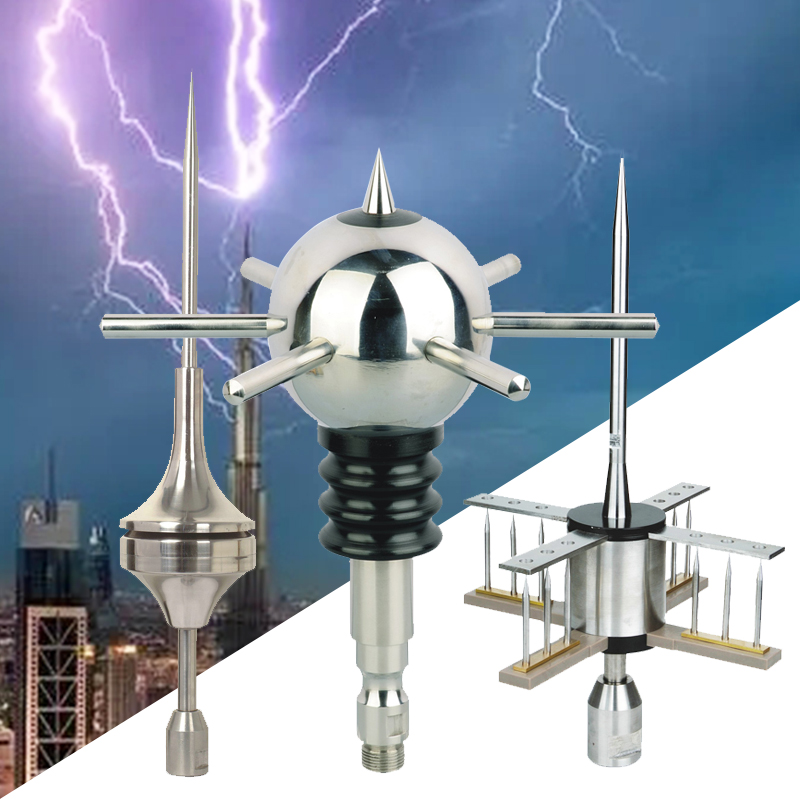The image displays an electrifying scene against a dark teal blue sky filled with jagged, illuminated purple lightning bolts. In the background, skyscrapers resembling space needles climb sharply into the stormy night, tapering off diagonally from the top right to the bottom left. Dominating the foreground, three intricate metal objects, reminiscent of industrial lightning rods, stand prominently. The structure on the far left features a slender top widening into a bell shape, while an inverse bell shape with an extended skinny piece adorns its other end. The central object showcases a spiked ball with six protrusions radiating outward, supported by a black cylindrical base and a silver stem. The rightmost piece presents a pointed rod at the top, transitioning into a spool-like middle section with four side arms, each hosting three nail-like appendages. These elaborate metallic forms align with the towering backdrop, suggesting a complex, high-tech urban installation designed to interact with the dramatic play of lightning in the sky.